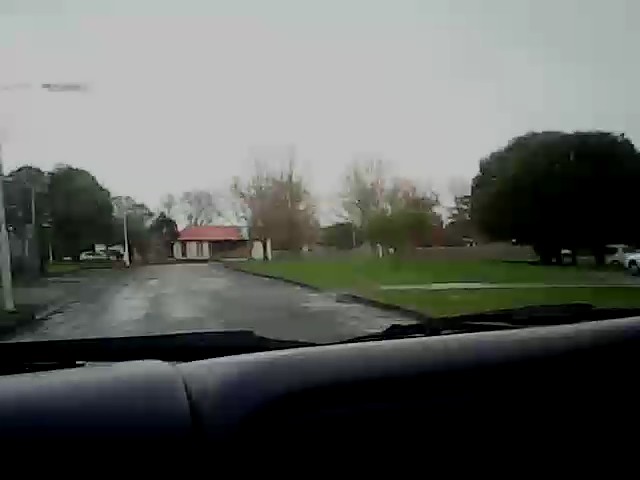Captured from the vantage point of a vehicle’s backseat, the bottom of this image features the top of the seat, creating a horizontal black band across the frame. Gazing out the window, the scene appears slightly blurry and veiled in an overcast haze, suggesting a rainy day. The road in the rearview glistens as if recently kissed by raindrops. To the right, a large grassy expanse showcases three distinct trees. The tree on the far right stands robust and lush, its dark green foliage forming a full, rounded canopy. In contrast, the two trees to its left are sparse and straggly, evoking a sense of barrenness. At the end of this wet, reflective road sits a building with tan walls and a prominent red roof, anchoring the scene with a touch of architectural presence.